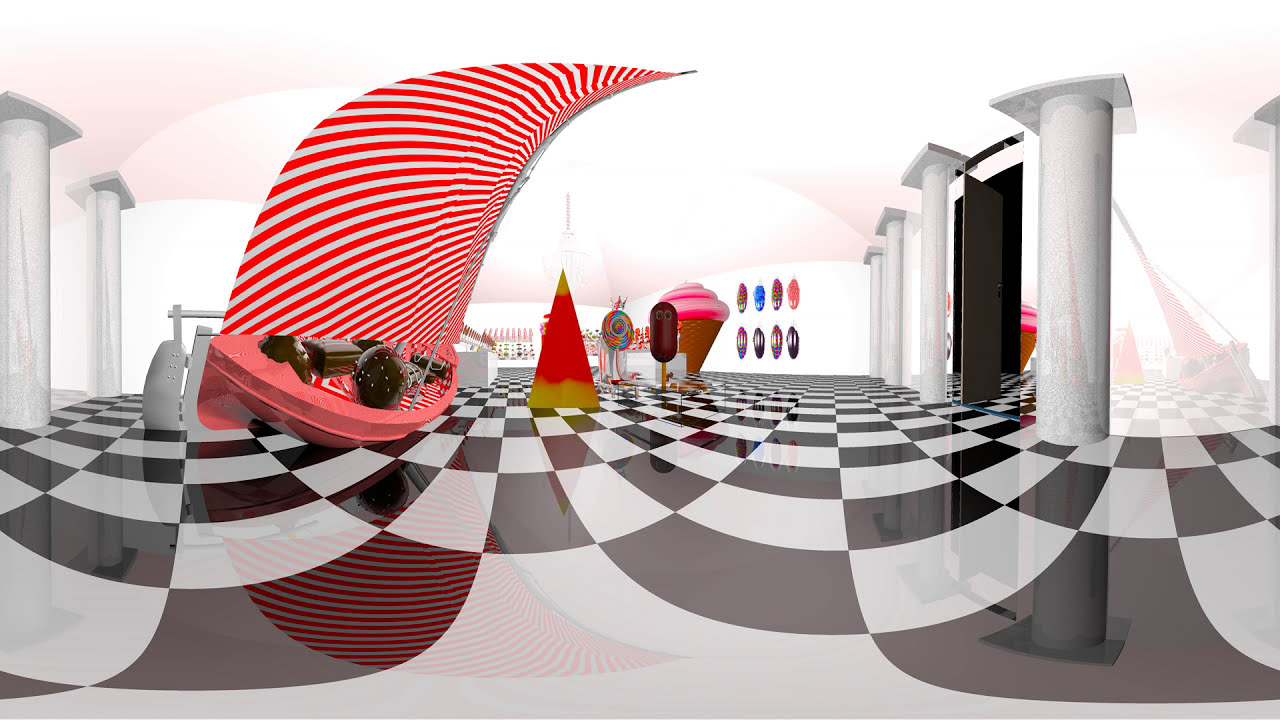The image is a computer-generated scene characterized by a highly reflective black and white checkerboard floor. The centerpiece is a whimsical, abstract sailboat with a red hull and horizontally striped red and white sail. The boat seems to be tilted on its side and includes brown elements resembling a chest and chairs. Flanking this scene, there are cylindrical white columns—two on the left and four on the right—whose images are also mirrored on the glossy floor.

Dominating the center of the composition is a giant candy corn standing upright with distinct yellow and orange sections. Nearby, a colorful swirl lollipop and a strange corn dog with eyeballs are prominently displayed. There’s also a large ice cream cone topped with what seems to be red ice cream.

On the back wall, several masks are arranged in a row, adding to the surreal environment. An open doorway between columns on the right reveals another room extending into the distance, which intriguingly appears to loop back, offering a reversed view of the sailboat. There are no visible markings or credits to indicate the creator or the source of the artwork.